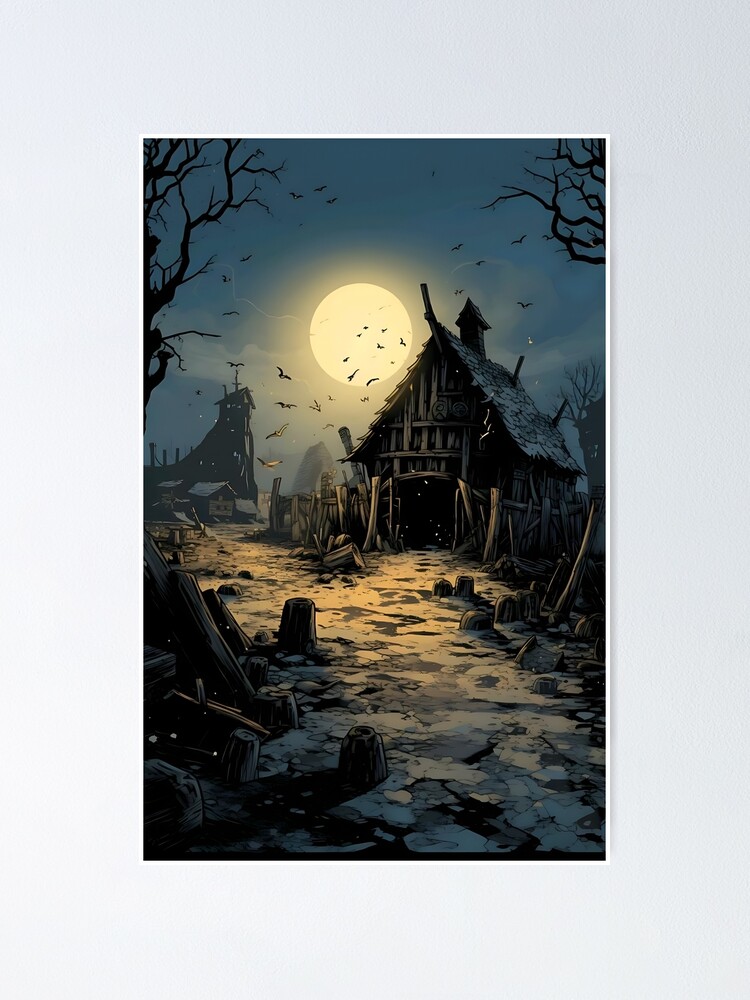This animated illustration portrays a nighttime scene dominated by a large, glowing full moon, which casts an ethereal light over the landscape. In the foreground stands a dilapidated barn, its structure barely holding together amidst a scattering of wooden planks. Two similarly ramshackle barns can be seen in the distance, adding to the sense of decay and abandonment. The night sky, dotted with a few sparse clouds, looms overhead, creating an eerie atmosphere. Birds are depicted in mid-flight, circling in various directions, adding a sense of movement to the otherwise still scene. Trees flank the barns on the left, right, and rear, their dark silhouettes blending into the misty air that permeates the area. The oversized moon dominates the background, its unusual size enhancing the surreal and haunting quality of the image.